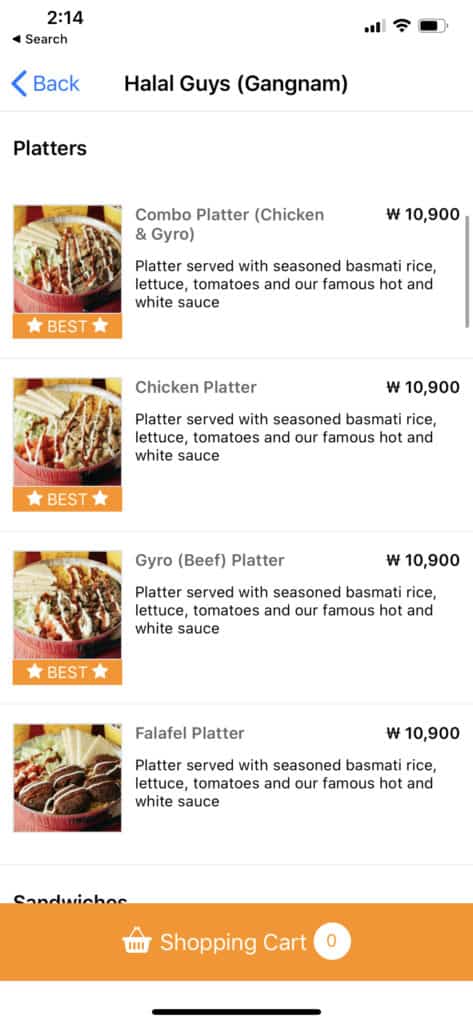This image depicts a white background with several elements arranged in a structured manner.

At the very top, there is a small text that reads "Search" accompanied by a left-pointing arrow. Above this section, in the top status bar, the time is displayed as "T14" on the left, while the right side shows the Wi-Fi signal icon, cell signal bars, and battery status icon.

Below the search area, a blue left-pointing arrow is labeled "Back" in blue text. Centered beneath this, the title "Halal Guys" is prominently displayed in capital letters. Following the title, "Gangnam" is enclosed in parentheses, also in capital letters.

A thin horizontal line separates the title section from the content below. The main content is divided into four sections:

1. **Combo Platter**: 
   - Described as "Chicken and Gyro".
   - Includes an image to the left.
   - An orange banner below the image reads "BEST" with white stars on each side and a caption that states "Why not eat both?"

2. **Chicken Platter**: 
   - Accompanied by an image.
   - Again, an orange banner beneath the image reads "BEST" with white stars on either side.

3. **Gyro (Beef) Platter**:
   - Paired with an image.
   - An orange banner beneath the image reads "BEST," flanked by white stars.

4. **Falafel Platter**:
   - Features a different image.
   - This section does not have the "BEST" banner.

At the bottom of the image, there is an orange banner displaying a shopping cart icon with the number "0" inside a circle, indicating an empty cart. On the opposite side of this banner, there is another shopping cart or basket icon.